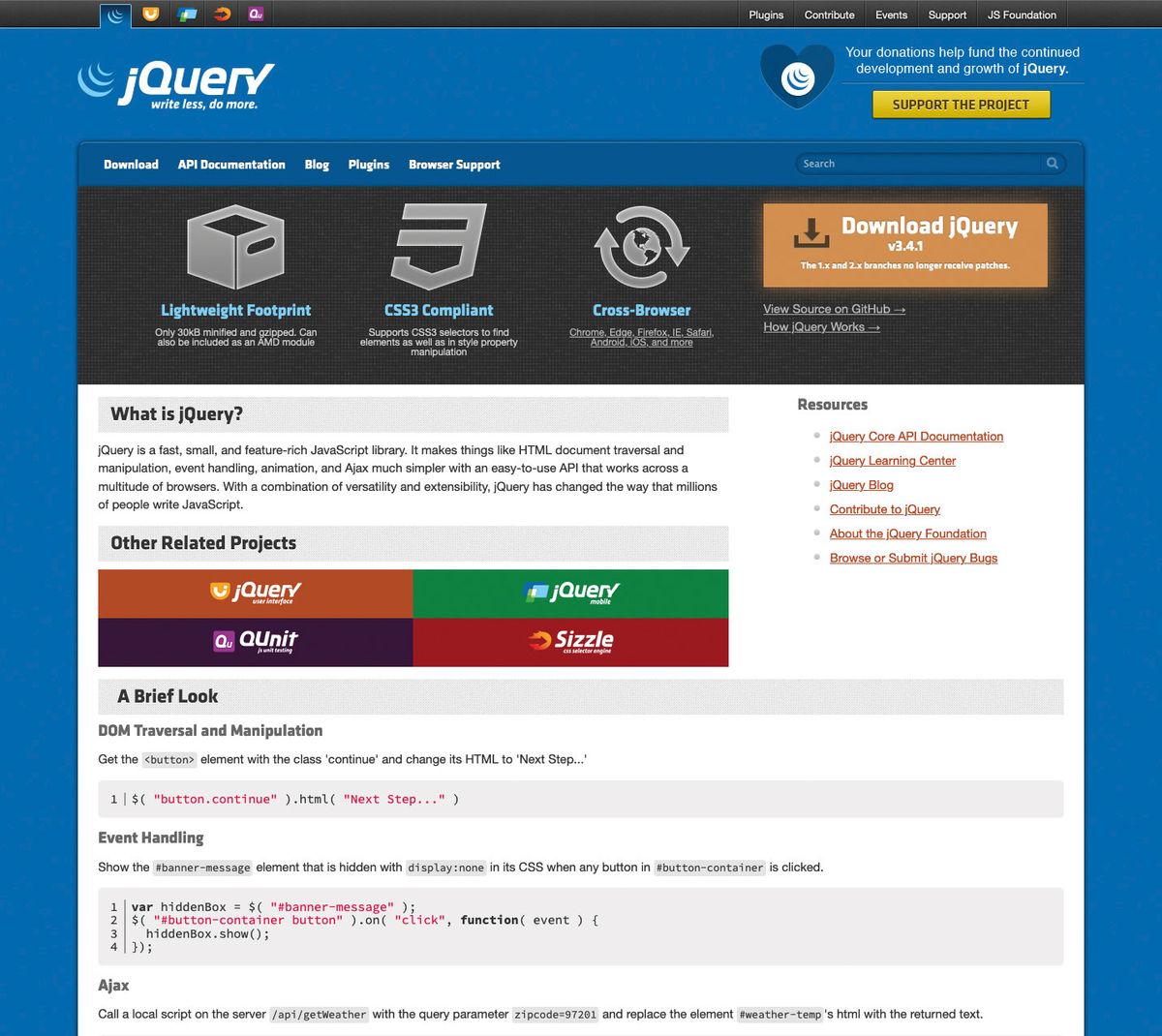**Detailed Caption:**

The image features a blue background with various elements laid out in a structured format. At the top, there is a prominent black box. Below it, a small blue tab with curved blue lines emerges, adjacent to a small brown element, a blue one, and an orange circle. A purple box is also present. 

At the very top, headers are visible, accentuated against the blue background, again featuring the characteristic blue swirly lines. The text "jQuery: Write Less, Do More" stands out, accompanied by a blue heart enclosed in a white circle adorned with blue lines. A message encourages donations to help fund the continued development and growth of jQuery. 

A yellow button labeled "Support the Project" prompts user interaction. Below this, there's a blue box offering options for "Download," "API Documentation," "Plugins," and "Browser Support," along with a search box.

Further down, a large black box showcases features like "Lightweight Footprint," "CSS3 Compliant," and "Cross-browser." Adjacent to this is a brown box with a dropdown labeled "Download jQuery Version 3.4.1" accompanied by a subtle white line underneath.

The image continues with a prominent white box detailing "What is jQuery," followed by explanatory text. Another blue box highlights "Other Related Projects," listing items such as a brown box for jQuery, a green box, a purple box for QUnit, and a red box for Sizzle.

Toward the bottom, a blue box titled "A Brief Look" describes aspects of "DOM Traversal and Manipulation," featuring a mini toolbar with icons for "one," a dollar sign, "button.continue," and "next step."

The section on "Event Handling" outlines four steps, some printed in red for emphasis. Lastly, a segment on "Ajax" discusses fetching a local script on the server, concluding the detailed overview.